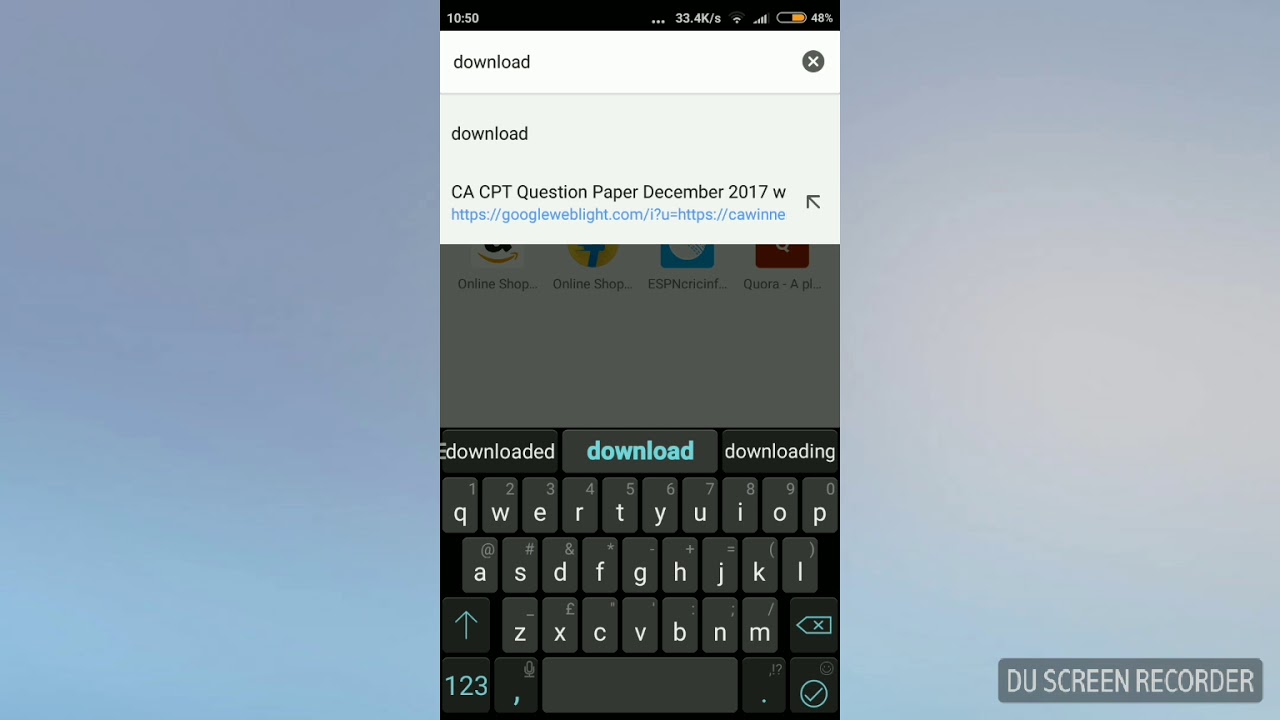In the image, a cell phone screen stands prominently against a dynamic and colorful background. The left side of the backdrop is predominantly bluish-gray, gradually transitioning to a mix of yellow, pink, green, gray, and blue hues towards the right. At the very bottom right-hand corner, a gray box with the label "DU Screen Recorder" is visible, indicating the method used to capture the screen image.

Focusing on the phone's screen in the center of the image, the time is displayed at the top within a black rectangle, reading "10:50." Adjacent to this, the Wi-Fi signal icon is displayed, followed by an indication that the battery is 48% full, with the battery icon filled in orange. Below these status indicators, there is a white region containing the text "Download CACT Question Paper, December 2017 W," accompanied by an HTTPS link for downloading the document.

As the eye moves further down the screen, the background shifts to a gray section leading to the phone's keyboard at the bottom, showcasing the typical layout for text input. Overall, the image captures the seamless blend of diverse colors in the background while detailing the elements visible on the cell phone screen.